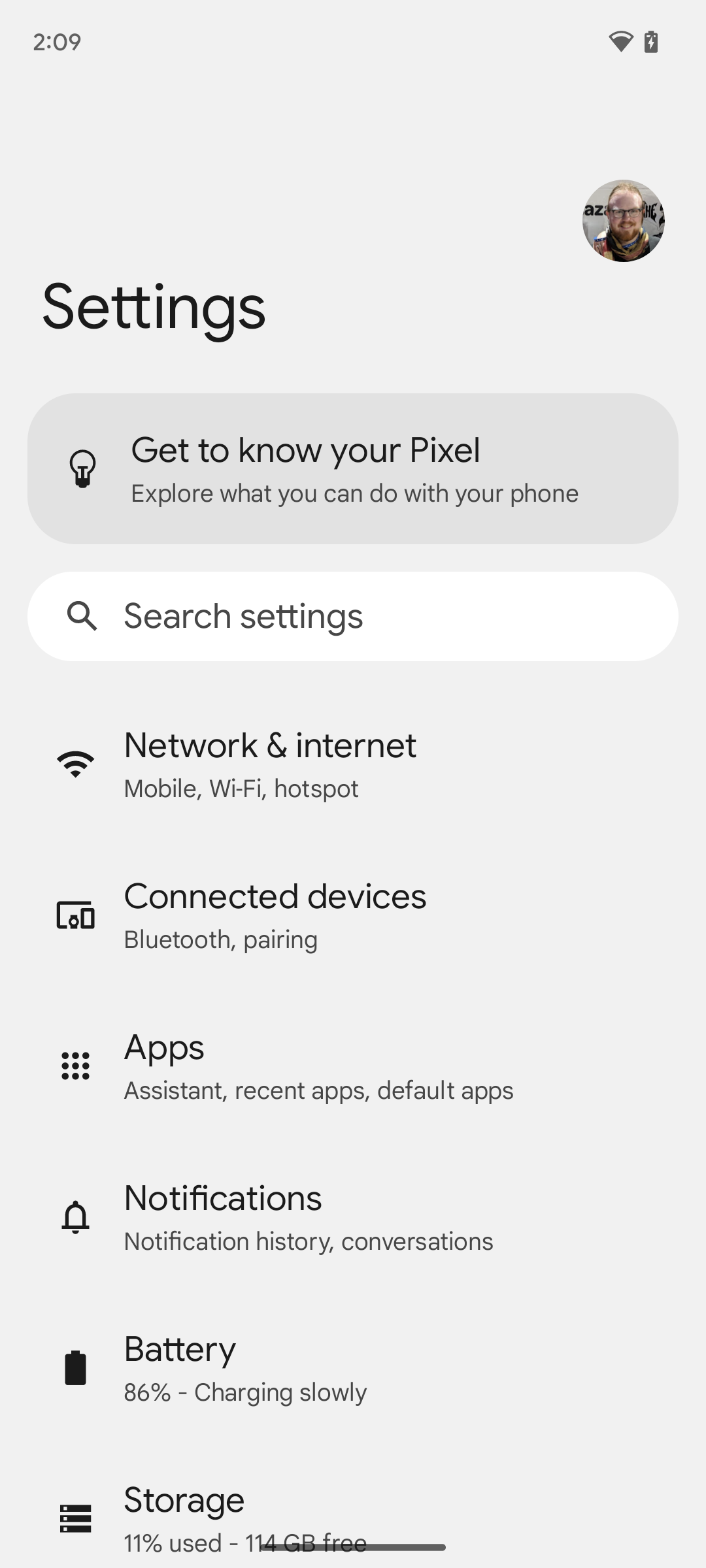The image displays a user interface from a Pixel smartphone's settings menu. At the top, a light gray rectangle features the number "209" alongside icons indicating Wi-Fi connectivity and battery status. Below this, a circular icon depicts a man's head. 

Following that, there's a "Settings" option and a gray, rounded rectangle with a light bulb icon on the left, labeled "Get to know your Pixel," which invites users to explore their phone's features. 

Another rectangular section bulges slightly on the sides, showcasing a magnifying glass icon on the left and the text "Search settings." Beneath this are various options organized into categories. 

First, a Wi-Fi symbol leads the "Network & Internet" section, which mentions mobile, Wi-Fi, and hotspot settings. Next, an icon resembling a partially outlined square with a circle and rectangle inside it is labeled "Connected devices," highlighting Bluetooth pairing. 

A square composed of dots denotes the "Apps" section, which includes information about the assistant, recent apps, and default apps. A bell icon introduces the "Notifications" area, covering notification history and conversations.

Further down, a battery icon indicates "Battery 86% - charging slowly." Below this, three vertically stacked rectangles with white dots symbolize the "Storage" section, showing "11% used," although the remaining text is obscured by a gray line, rendering it unreadable.